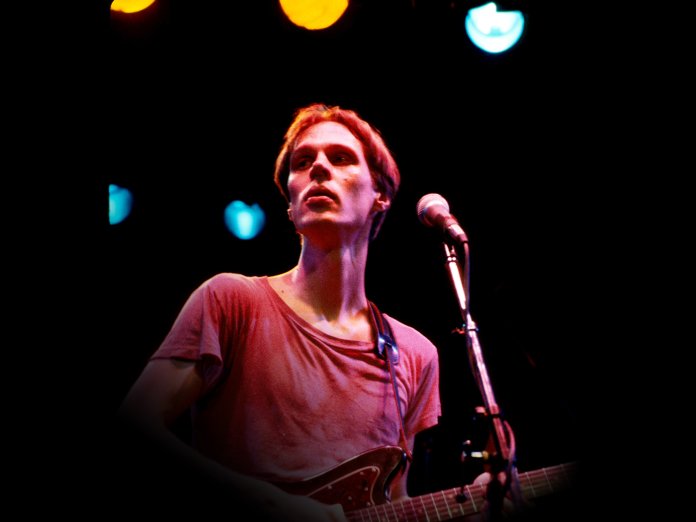The image captures a live performance scene featuring a slim male musician on stage, framed from the waist up. He dons a faded red short-sleeve shirt, which appears slightly worn. His short, shaggy brown hair is highlighted by the stage lighting, casting a yellow hue, particularly on his hair, giving him a slightly redder appearance than normal. The musician, who has a pronounced jawline, gazes thoughtfully towards the upper left. He cradles a black electric guitar, held by a strap over his right shoulder, with one hand positioned on the strings. A corded microphone stand ascends diagonally from his bottom right towards his face, placed in front of him. The stage behind him is enveloped in pitch black, accentuating the vibrant stage lights. Above his left shoulder are several blue and yellow spotlights, including a semicircle of yellow light and another of blue in the middle top section of the image, while additional blue lights glimmer further to the left. The overall lighting and positioning suggest a dynamic and moody atmosphere, captured from slightly below stage level, looking up at the performer.